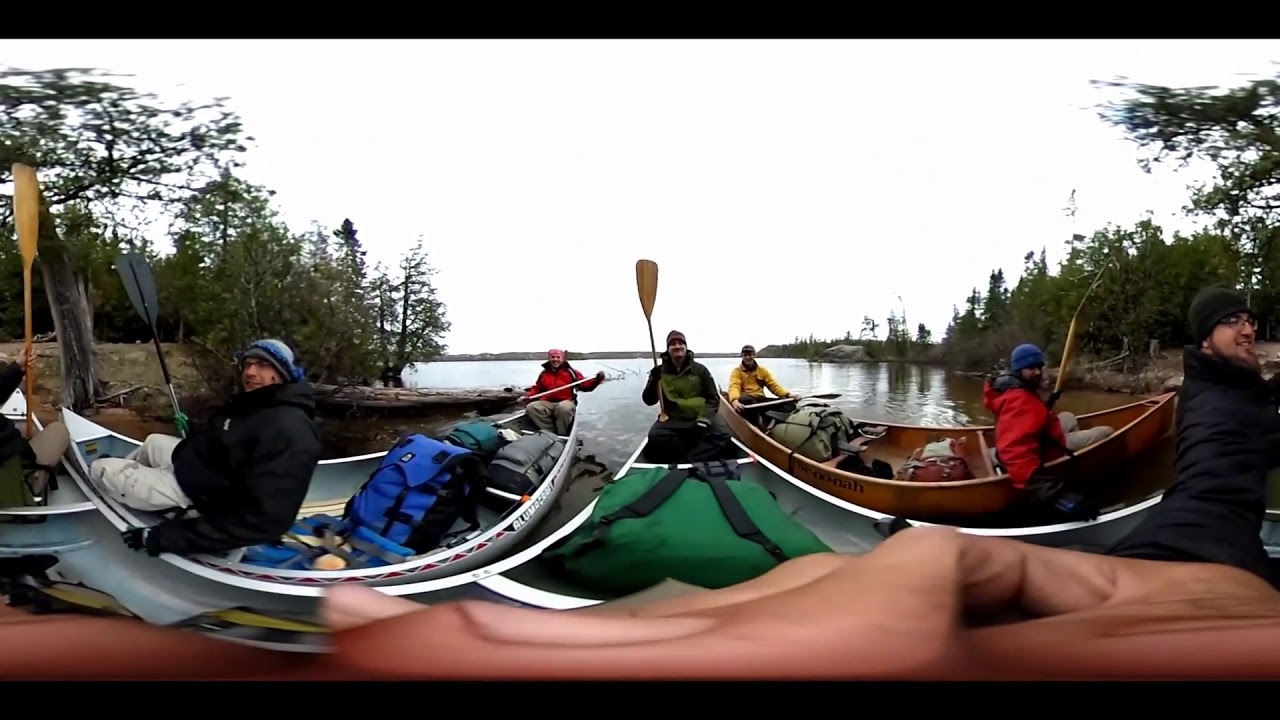In this selfie, a group of six people is captured on a somber day of canoeing or kayaking. They are spread across three boats on a lake or river, positioned near the shore rather than deep in the water. The individuals are dressed warmly, suggesting it's fall, as they sport winter caps and jackets. The man taking the selfie is wearing a black jacket and hat. In the other boats, one person is in a red jacket and blue hat, another in a green jacket, one in a yellow jacket, another in a red jacket, and a final person in a black jacket and blue-and-light-blue hat. Notably, three men are raising their paddles in the air while two hold them straight across. The boats differ in color, with at least one being white and another brown. Visible in the background are some green elements, juxtaposed against the predominantly gray day, adding to the sense of a brisk outdoor adventure.